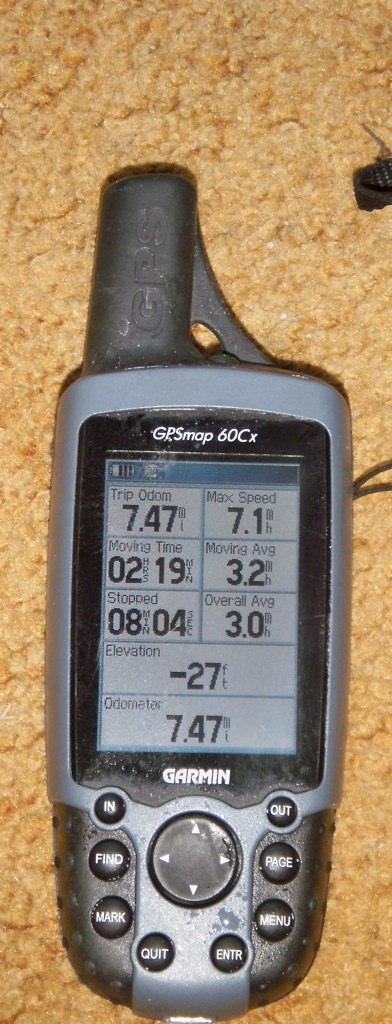The photograph showcases an antique GPS tracking device resting on a textured, brownish wool-like carpet. The carpet, resembling thick oatmeal in its texture, provides a rustic backdrop to the device. The GPS tracker, visibly aged and slightly worn, features a small black handle at the top made from a rubber-plastic material, labeled "GPS." Shaped similarly to a cell phone, the device has a sturdy gray metal perimeter. The top of the device bears the model name "GPSmap 60C," and the screen displays various measurements such as "trip odometer 7.47," "max speed 7.1," "moving time 02:19," "moving average 3.2," "stopped 08:04," "overall average 3.0," "elevation -27," and "odometer 7.47." The renowned brand "Garmin" is prominently displayed in white text below the screen. The lower section of the device is equipped with a black directional button surrounded by multiple smaller black buttons in a U-shaped layout, labeled with functions such as "in," "find," "mark," "quit," "enter," "menu," "page," and "out."